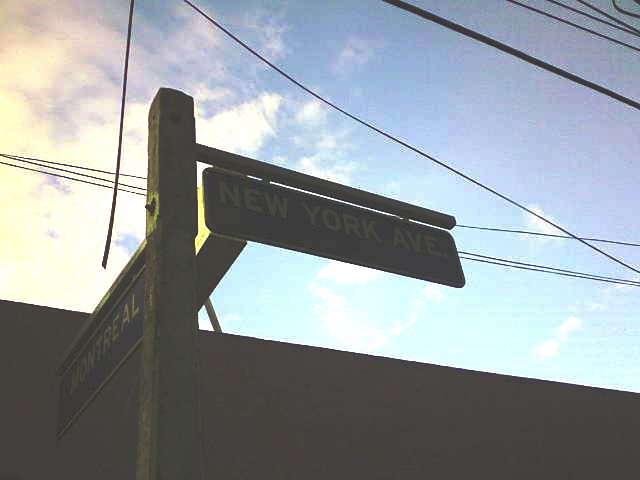This evocative painting captures a nostalgic cityscape with striking details. The scene is dominated by a wooden post with two perpendicular street signs, signaling New York Avenue on the right and Montreal on the left, both in white letters on black backgrounds. The perspective is from below, giving a clear, upward view of the power lines crisscrossing the top of the image, one visibly dangling loosely. The sky serves as a vivid backdrop with its stunning palette of pastel hues—ranging from a bluish tint at the bottom middle to darker bluish-purple on the top right, complemented by a pinkish-purplish glow in the top left. Bright, white clouds gather on the far left, hinting at the sun's hidden presence. Silhouetted against the lower portion of the sky, a dark building's outline subtly grounds the otherwise airy scene, enriching the composition with its enigmatic presence.